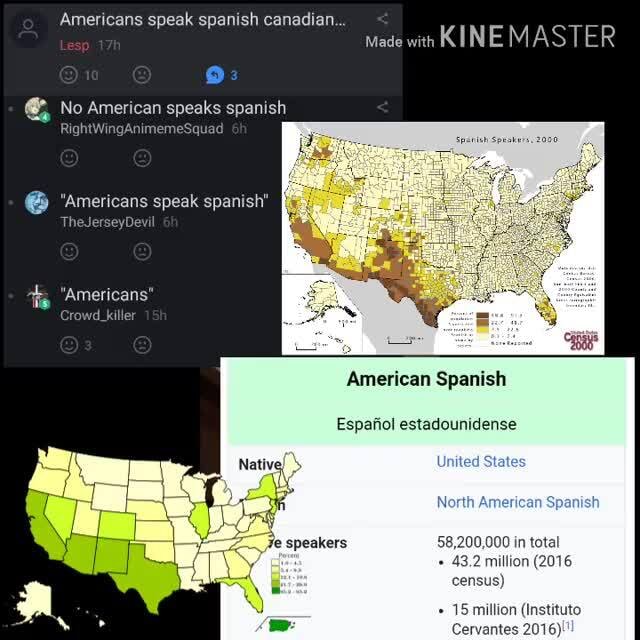Here is the refined and detailed caption for the image:

"This image is a screenshot made with KineMaster, featuring two maps of the United States of America. The first map displays the geographic distribution and concentration of Spanish speakers in the year 2000, using dark brown to indicate the highest number of Spanish speakers and white to indicate the lowest. The data originates from the Census 2000. Additionally, the image includes information about American Spanish, highlighting that there were 58.2 million Spanish speakers in total. According to the 2016 Census, this number was 43.2 million. The image also contains comments emphasizing that a significant number of Americans speak Spanish."